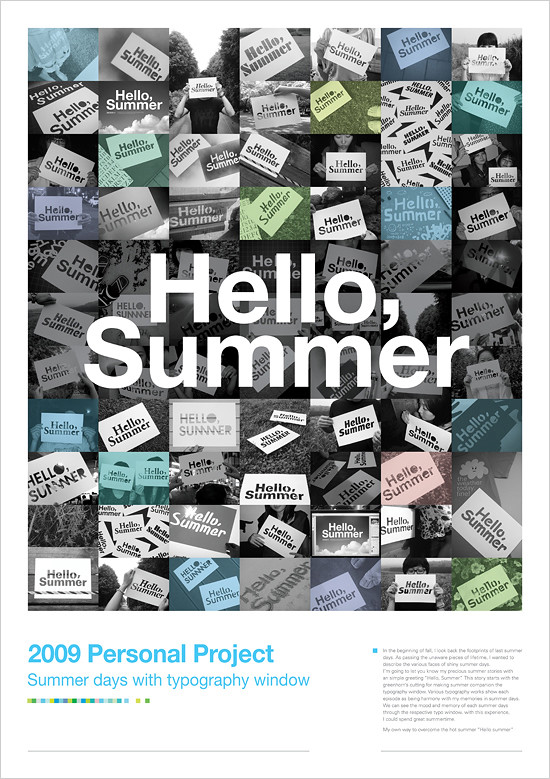This is a photograph of a vertically-oriented white poster. The top section of the poster features a collage of 77 smaller rectangular images arranged in a 7x11 grid. Each image showcases the phrase "Hello Summer" displayed in various fonts and styles. Some images feature people holding signs, some have the phrase written against different backgrounds, such as a sky with clouds, and others use a mix of black, white, turquoise, light blue, and multiple color schemes. The central part of the collage prominently highlights "Hello, Summer" in white text.

The lower third of the poster contains additional text elements. On the bottom left, in a turquoise color, it states "2009 Personal Project Summer Days with Typography Window." To the right, there's a block of smaller text, which is mostly unreadable due to the small font size. The bottom section also includes several colored squares aligned in a row, featuring shades of light and dark green, white, and blue, adding to the poster’s overall visual diversity.